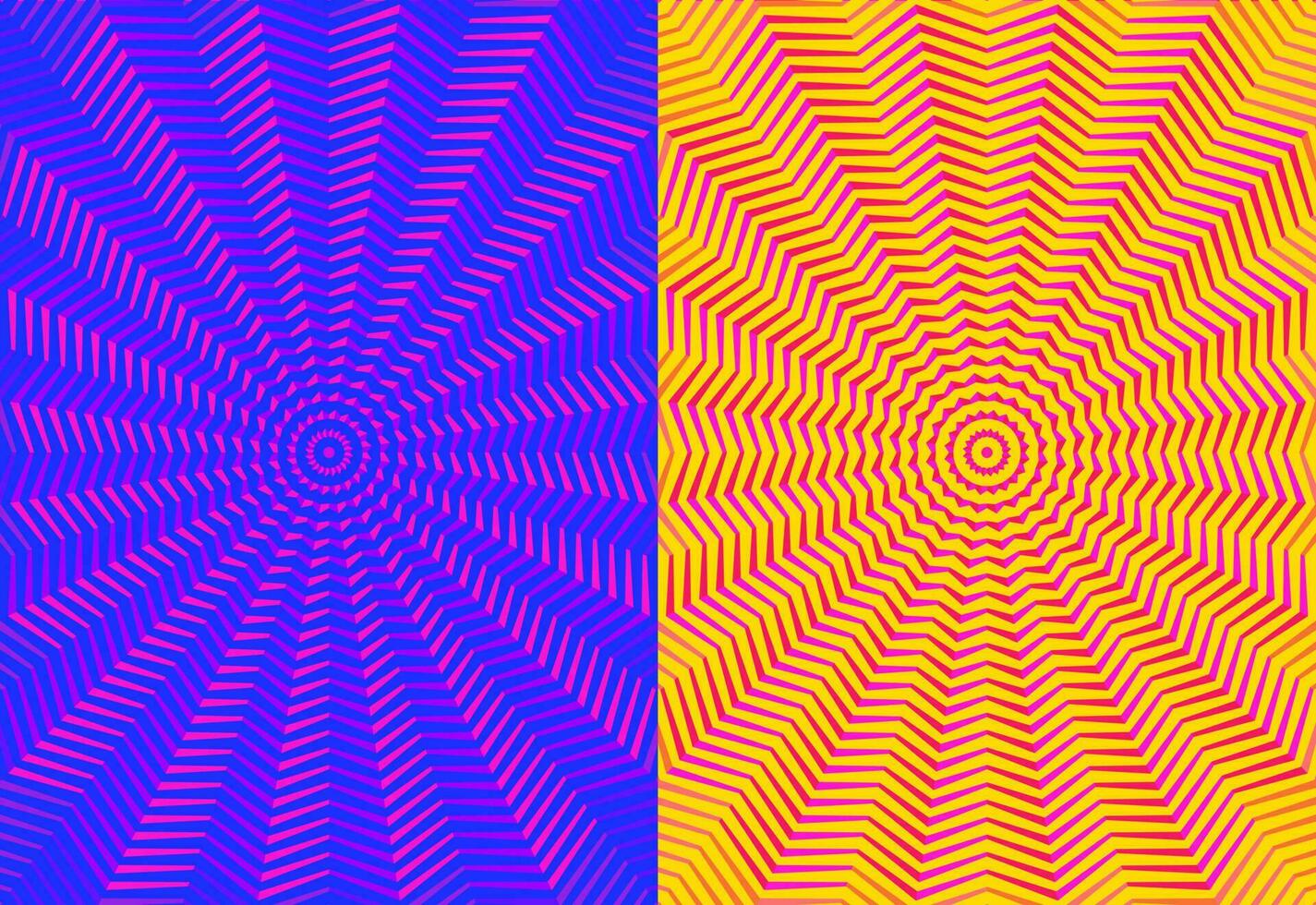This double-sided large square poster features two adjacent digital illustrations, exuding a strong psychedelic vibe. Both halves showcase the same geometric pattern arranged in a spiral, radiating from a central circle outwards with an optical illusion effect. The left side is adorned with a pink spiral on a blue background, while the right mirrors this pattern but employs a yellow background with red lines. The intricate design consists of long, rectangular sun rays or jagged, triangular ridges unfanning from the central spiral, creating a sense of depth and motion as though the spirals are spinning, further emphasized by the boldness of the yellow and red colors compared to the slightly muted blue and pink. This visual interplay of undulating lines and vibrant colors connects seamlessly at the center, enhancing the overall dynamic and mesmerizing impression that shifts as one continues to gaze at it.